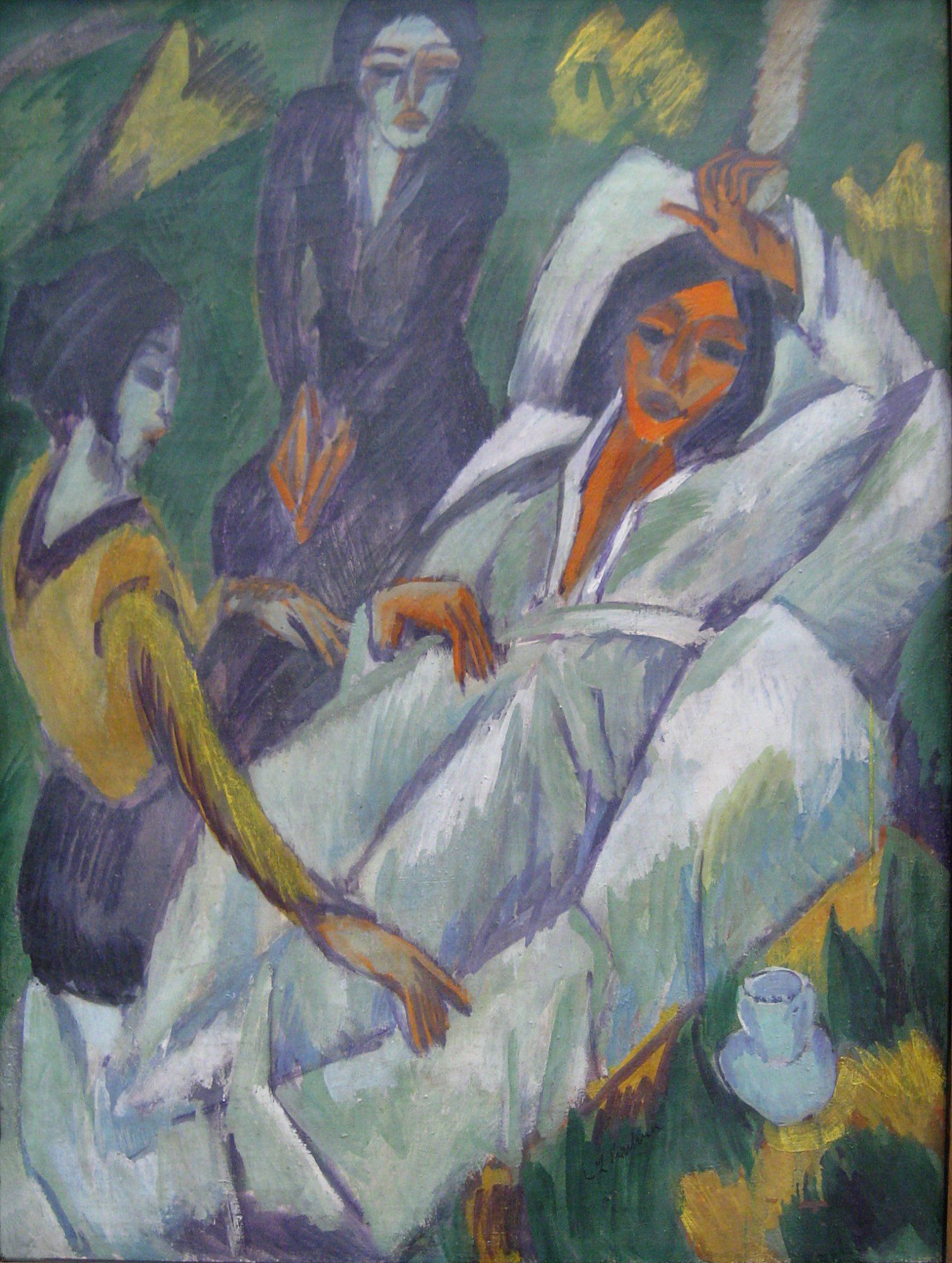This vertically oriented Impressionist artwork, likely from the early 1900s, depicts a scene featuring three women. The central figure, a dark-haired woman adorned in a white robe, is reclining on a white cushion or sofa. She appears to be in a state of repose, with one hand resting on her stomach and the other on top of her head. Her skin has an orange hue, possibly suggesting illness or symbolic of a deeper theme. Nearby, a cup and saucer rest, adding a domestic touch to the scene.

Surrounding this central figure are two other women whose features and attire contrast with her. One woman, dressed in a dark suit with trim hair and red lips, sits by the head of the reclining woman, hands folded in her lap, gazing downward. The other stands by the reclining woman's feet, wearing a yellow long-sleeve shirt and dark pants or a skirt; her arm stretches protectively across the reclining woman's legs, which are concealed by the robe. The background features indistinct green and yellow shades, possibly grass or flowers, enhancing the surreal and dreamlike atmosphere of the scene. An unreadable artist's signature is present below the central figure, grounding the mysterious and evocative composition in the realm of fine art.